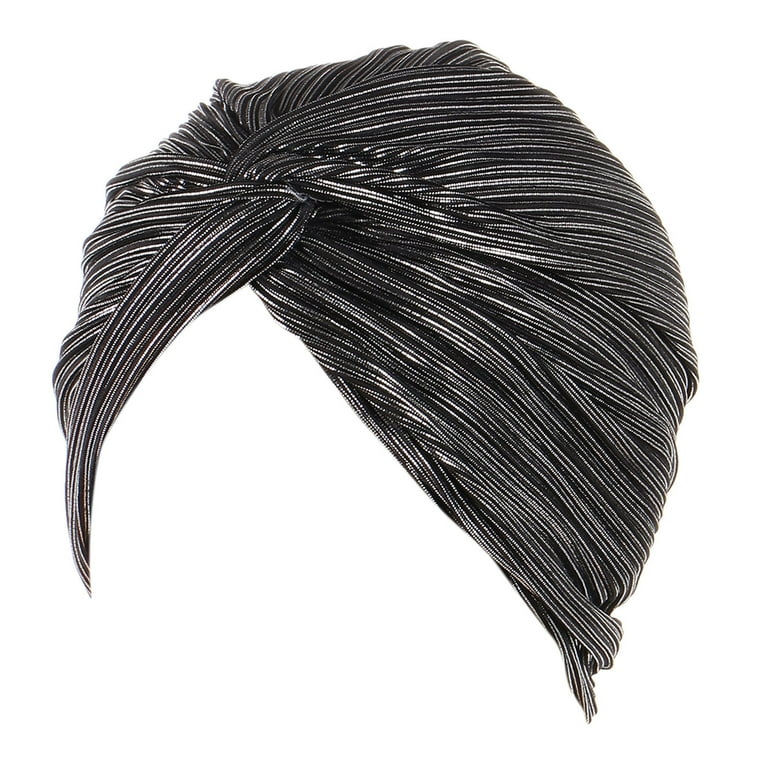This image depicts a photorealistic depiction of a traditional head wrap, often associated with African-American fashion, featured against a completely white background. The head wrap, crafted from a fabric displaying black, gray, and metallic silver pinstripes, evokes a metallic, wiry texture. It is knotted at the center of the forehead and extends around the head to where the base of the neck would be, covering the hair and ears while leaving the face area open. The intricate design, with its tight pinstripes and rounded form at the top, suggests it could be part of a catalog or online store entry, presented with no face or body, enhancing focus solely on the head wrap's sophisticated appearance.